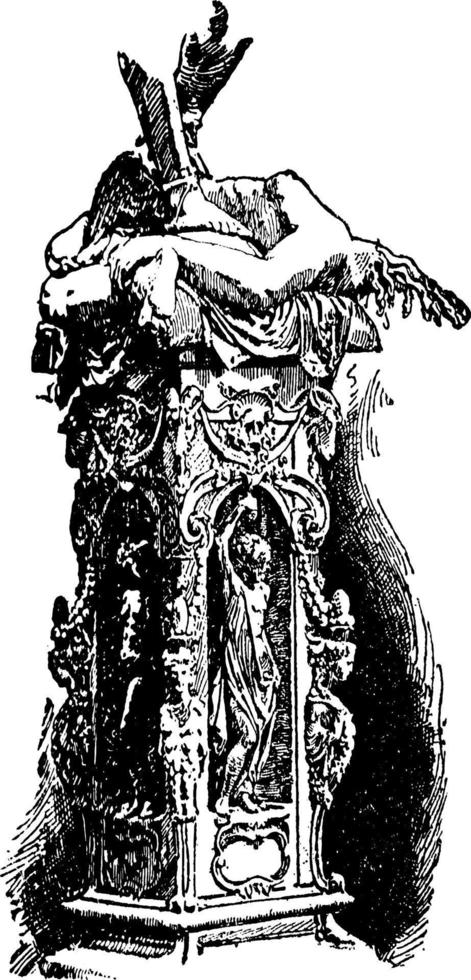This detailed black and white drawing depicts a tall, vertically oriented statue that gives the impression of a clock tower, heavily adorned with intricate design elements. The central focus is a nude figure with draped clothing, standing with their right arm raised. The statue, portrayed with significant shadowing and a Gothic-inspired aesthetic, features elaborate carvings on its sides, each corner detailed with human heads. Beneath the main figure, there's a circular area that appears reserved for a plaque or nameplate. Surrounding the central figure are curved lines adding to the complexity of the design, while the top is adorned with shapes resembling tree roots, adding to the overall dark and ornate atmosphere of the drawing. The composition lacks a border or background, making the statue appear to float against a stark white backdrop.